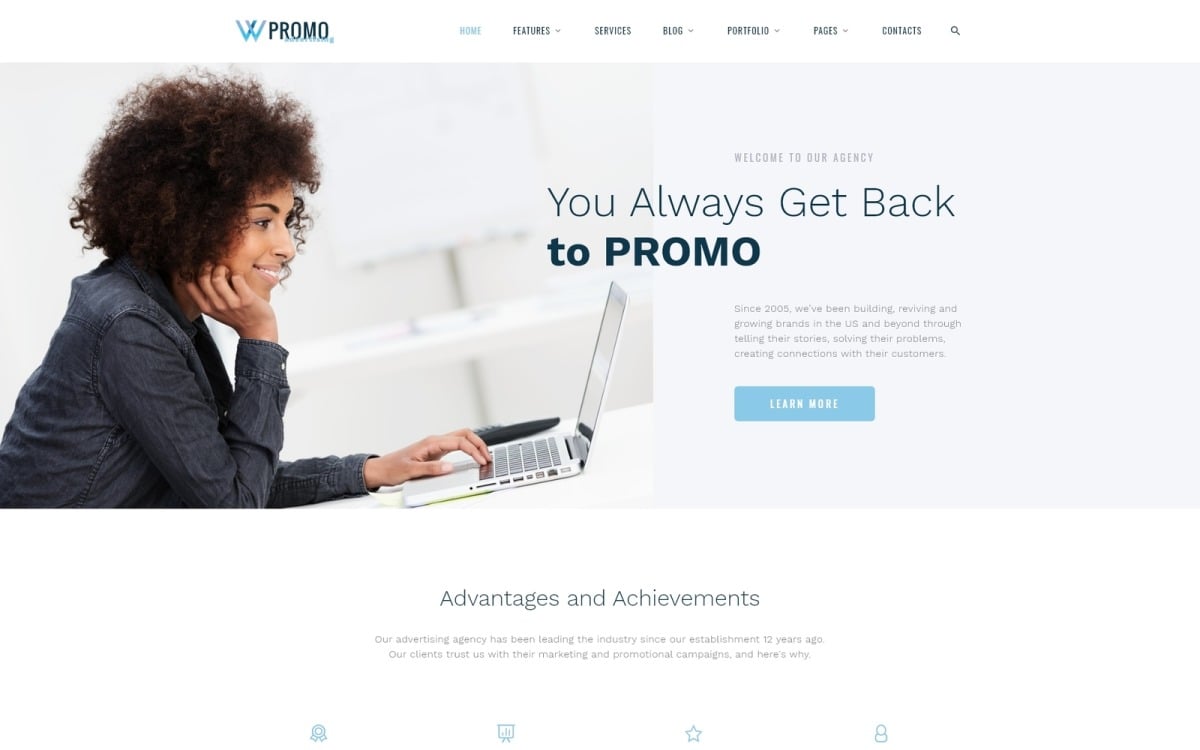This image is a screenshot from a computer or a phone displaying a web page. At the top left corner, the webpage title "WChrome" is prominently displayed. Adjacent to the title, we see the navigation menu items: "Features" in black letters, followed by "Services," "Blog," and "Contents," each separated by ample space. On the far right of the navigation bar, there's a magnifying glass icon indicating a search function.

Below the navigation bar, the main content of the screenshot includes a distinct gray shaded box contrasting slightly with the white background above. Inside this box, on the left-hand side, there is a woman sitting at a table engaged in work on her laptop. The laptop is open, and her left hand is positioned on the keyboard while her right hand is bent under her chin, possibly indicating a thoughtful or focused expression. The woman has brown curly hair and black eyebrows, and she is smiling, revealing her white teeth. She is dressed in a gray shirt or blouse with long sleeves, featuring white buttons on the cuffs.